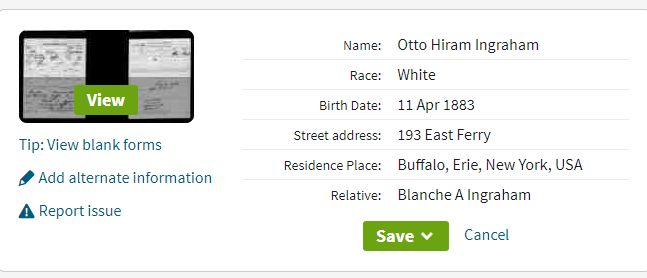The image features a digital form with light gray borders at the top and bottom. On the left side of the image, there appears to be a representation of two cell phone screens or sections of one, separated by a black outline. These screens have a black space between them and display some text. In the green box between the screens, the word "View" is written in white letters. Below it, the text reads: "Tip: View blank forms," followed by "Add alternate information," and "Report issue."

On the right side of the image, detailed biographical information about a person named Otto Hiram Ingram is listed. The details include:

- Name: Otto Hiram Ingram
- Race: White
- Birth Date: 11 April 1883
- Street Address: 193 East Ferry
- Residence Place: Buffalo, Erie, New York, USA
- Relative: Blanche A. Ingram

At the bottom right of the biographical section, there are two buttons: a green "Save" button and a "Cancel" button next to it. The layout and features suggest that this image is a screenshot of an informational sheet or form viewable on a computer, which likely allows users to interact with and edit the provided information.